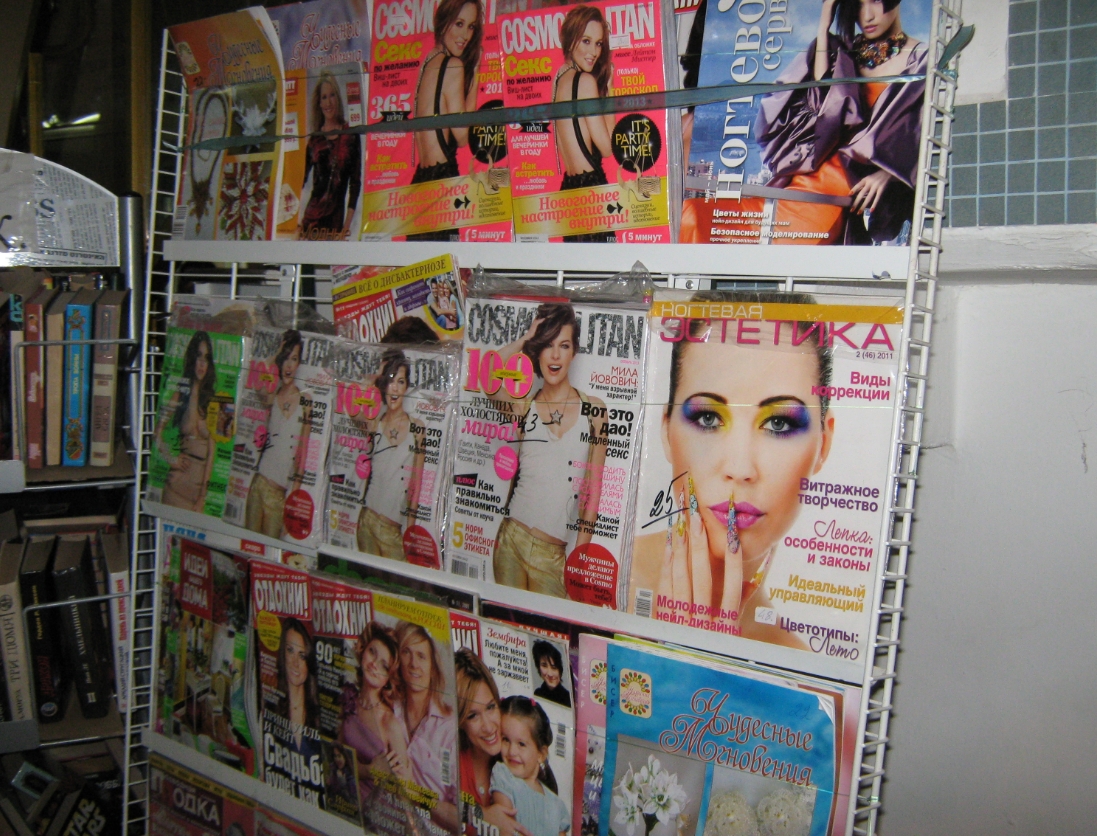The photo showcases a white wire magazine rack positioned against a white wall in a small store. The rack features four rows of magazines, prominently displaying an assortment of fashion and gossip publications. At the top row, there are pink Cosmopolitan magazines featuring a woman posing in the center. The next row houses three Cosmopolitan magazines with a different woman on the cover, in white. Some of the magazines have Russian text, hinting at an international selection. To the left of the magazine rack stands a silver book cart with a silver placard, displaying various books, including a visibly marked "Star Wars" book. Behind the rack, the white wall transitions to a gray, square, grid-like patterned section, possibly a board or window that is shining light into the room. There's also a suggestion of a ladder in the background, indicating the store might be in the process of closing or is generally a small, functional area.